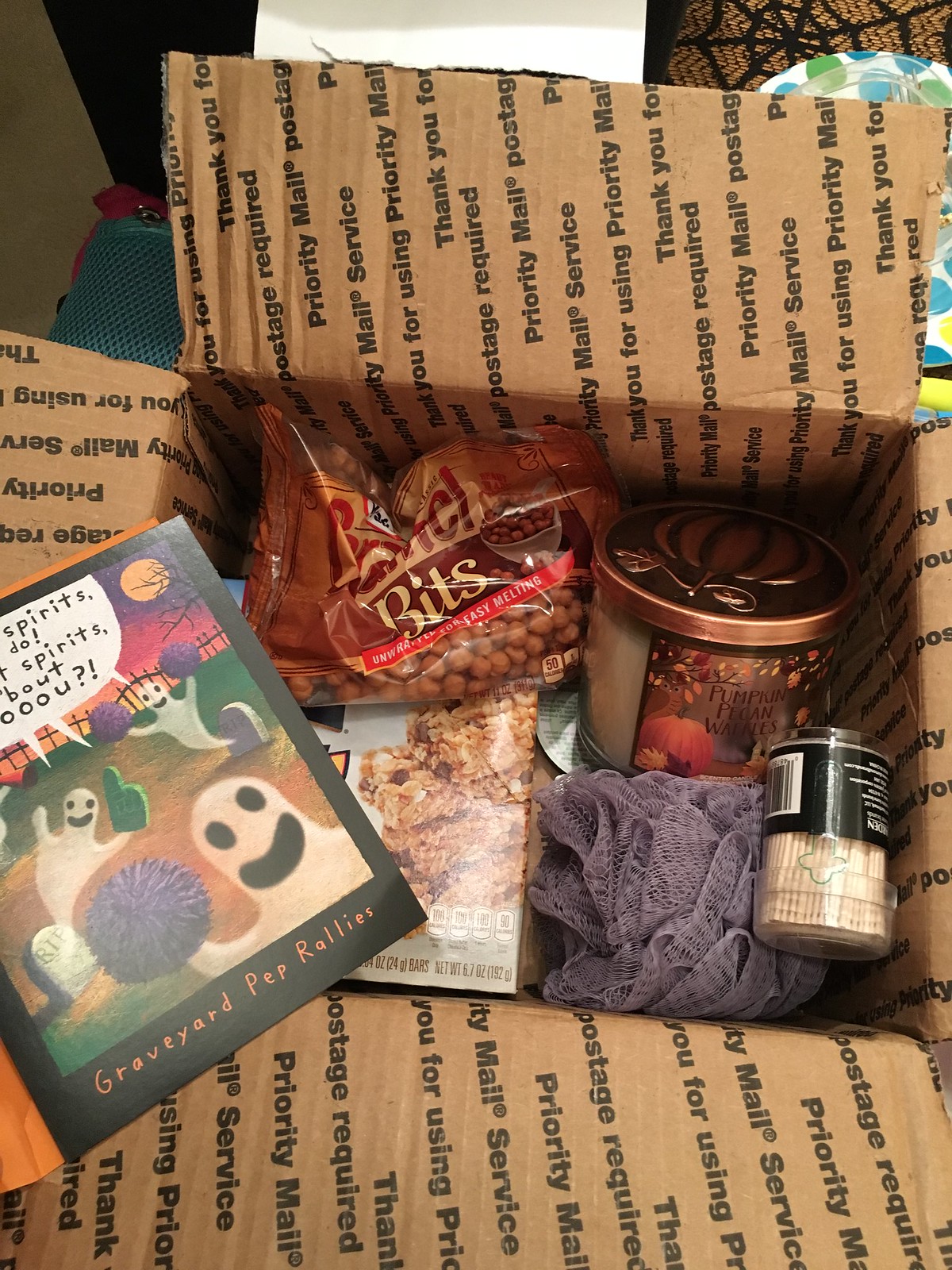The image depicts an open cardboard box labeled "Priority Mail" with printed text thanking the user for using Priority Mail Services. Inside the box, there is an assortment of items arranged carefully. At the forefront, a card featuring ghosts and the text "Graveyard Pep Rallies" is prominently displayed. Among the items, there's a bag of Caramel Bits and a pumpkin-scented candle labeled "Pumpkin Pecan Waffle" to the right. Positioned slightly beneath, there is a box of granola bars partially obscured by the card. Adjacent to this, a gray body loofah and a plastic container of toothpicks are visible. The detailed arrangement of the various items suggests a thoughtfully curated package.